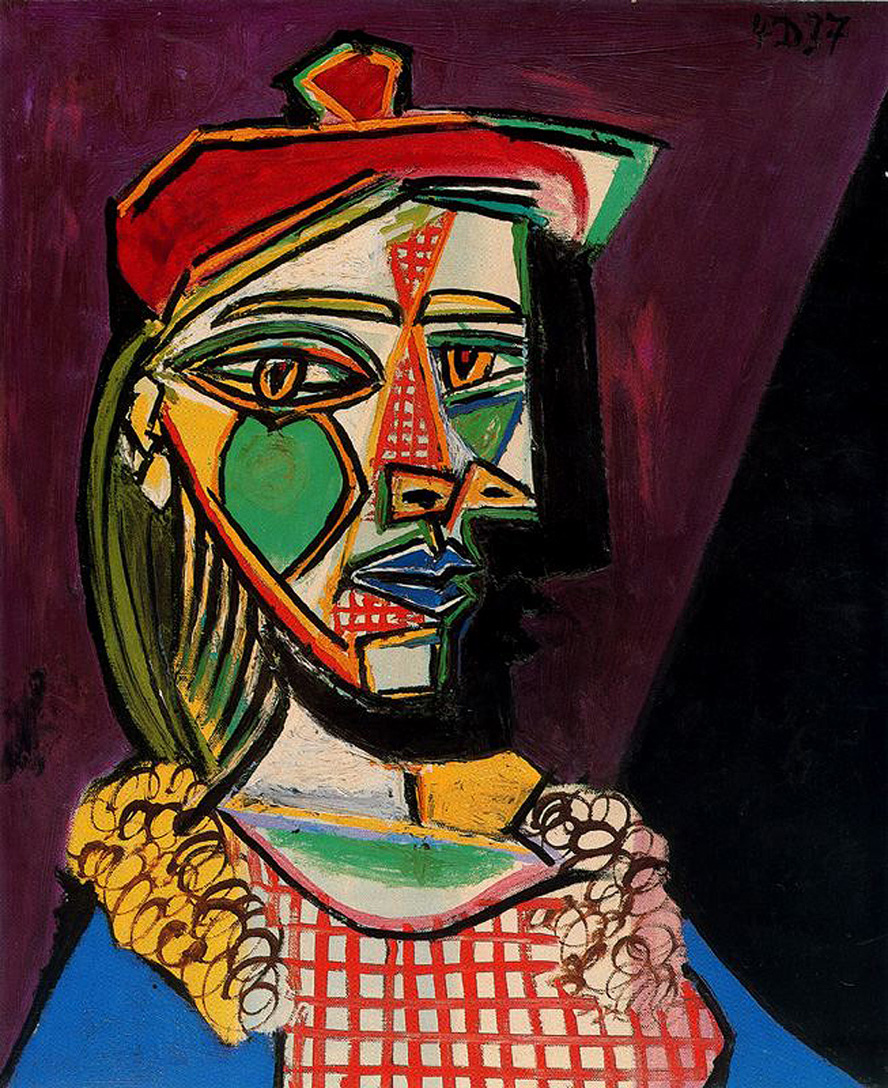The painting titled "Woman in Beret and Czech Dress" by Pablo Picasso showcases an abstract representation of a woman facing forward, characterized by Picasso's signature geometric and colorful style. The woman dons a red beret with a ball on top and her face is outlined with a thick black line on the right side. Her features are strikingly abstract; she has yellow-orange eyes, with the left eye larger than the right, and a nose that juts out geometrically. Her blue lips are sharply defined, and her cheeks are painted green, one triangular and the other circular. Her chin is shaped like a square or trapezoid, and her neck displays vertical stripes. 

She wears a blue shirt under a red checkered jumper with white details reminiscent of a Czech apron. Her arms extend to each side, covered in bright blue sleeves. Her hair falls in swirly black lines, colored yellow on the left and white on the right. The background is an angular deep plum interspersed with black on the right, with bursts of color, including yellow, olive green, tan, red, white, brown, and light purple accents around her neck. The painting's vivid and structured composition highlights primary colors, blending them into a harmonious visual experience that epitomizes Picasso's abstract style.